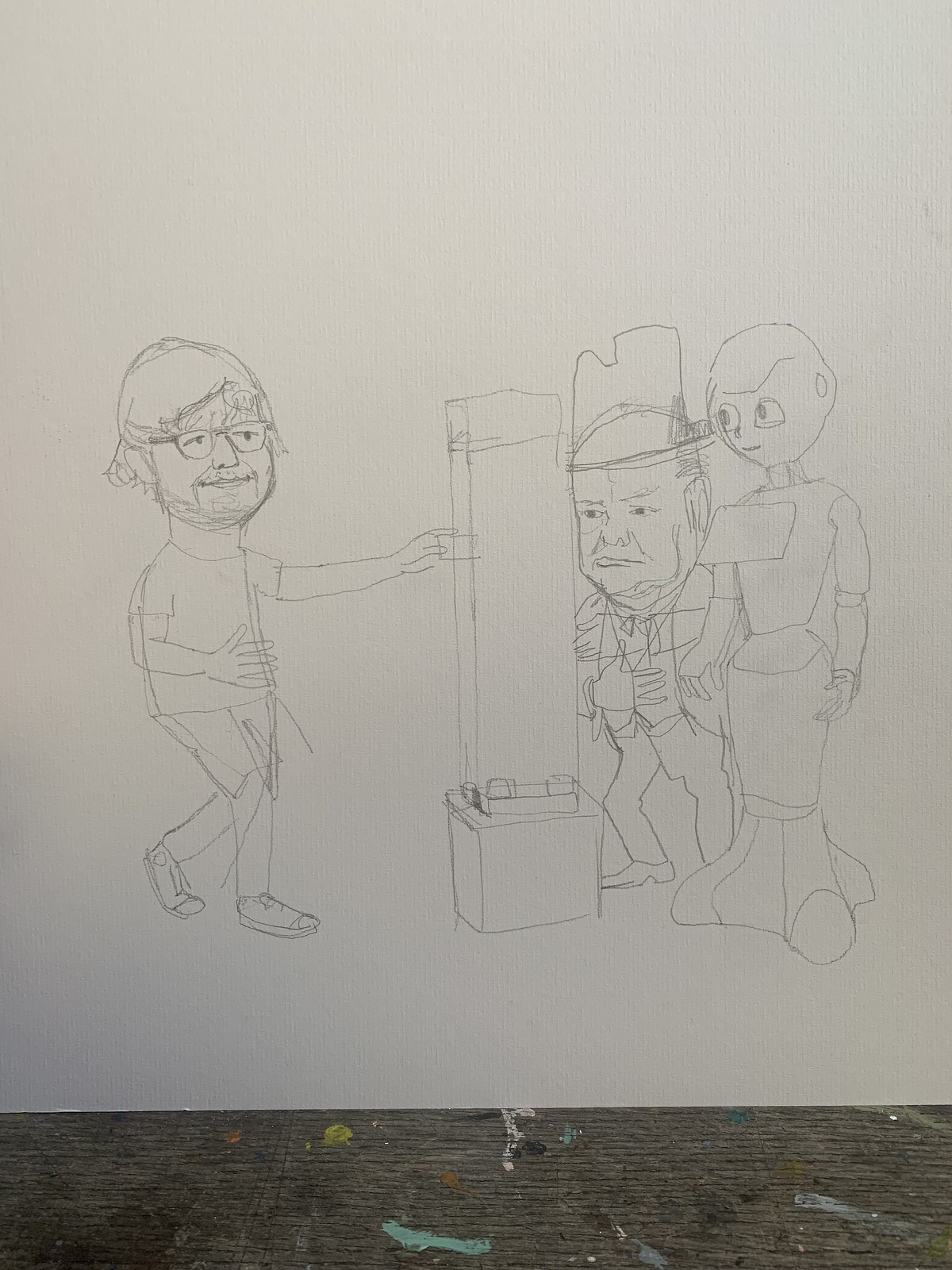This detailed pencil sketch, drawn on a clean white piece of paper and set against a gray wooden backdrop marked with various paint stains, depicts a scene blending caricature and comic book styles. The central figure on the left resembles Ed Sheeran, identifiable by his glasses, scruffy beard, short-sleeved t-shirt, pants, and shoes. He is interacting with a tall column-like object, possibly a ticket machine or water cooler, by pointing or placing something into it.

To the right of this machine stands an older, chubby man strongly reminiscent of Winston Churchill. He is dressed in a suit and a top hat, with prominent jowls defining his face. Next to him, there is a unique robot characterized by a round head displaying human-like facial features. The robot's body, shaped like a mechanical dress or gown with a solid base, adds a futuristic touch to the scene. The image contains no text to clarify the narrative, leaving the interaction between the man, the machine, Winston Churchill, and the robot open to interpretation.